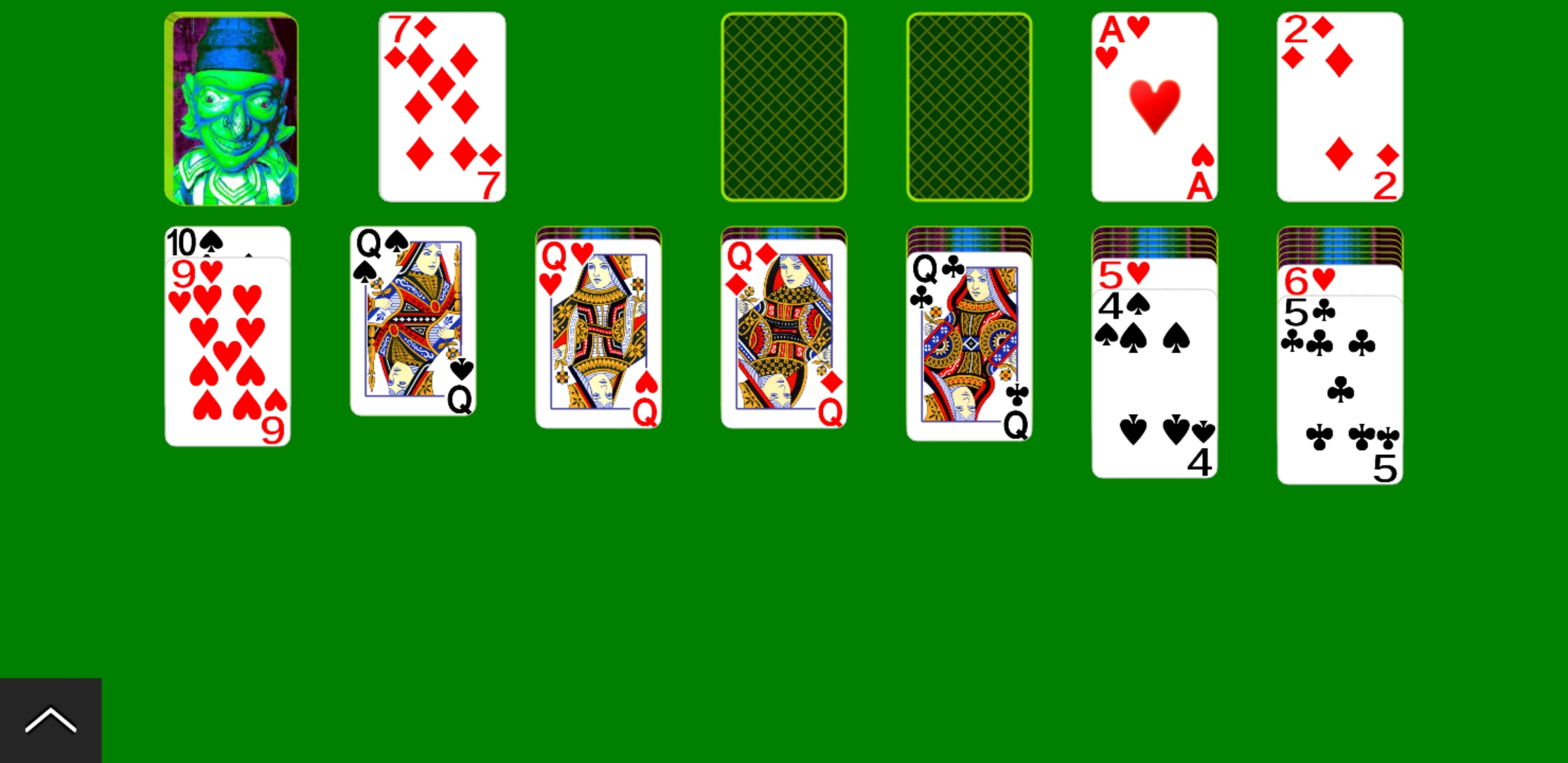The image depicts a solitaire game interface displayed on a rectangular screen oriented from left to right. The background boasts a dark grass green color with a hint of yellow, appearing smooth and flat without any noticeable texture or color variations.

At the top left corner, a deck of cards features an interesting character design: the card's background is purple, showcasing a green-faced figure adorned with a blue hat and blue markings around his eyes. He is dressed in a white, green, and blue outfit.

Directly below the deck, the visible tableau includes:

- A black Ten of Spades with a Nine of Hearts beneath it.
- A selectable Seven of Diamonds card positioned to the right of the deck.
- Adjacent to the Ten of Spades, there's a Queen of Spades.

The tableau also contains:
- A Queen of Hearts
- A Queen of Diamonds
- A Queen of Clubs
- A Five of Hearts
- A Four of Spades
- A Six of Hearts
- A Five of Clubs

Except for the Ten of Spades and Queen of Spades, each of these cards has multiple cards beneath it, not visible in the image.

At the top, the foundation piles intended for building ascending sequences show only an Ace of Hearts and a Two of Diamonds, with two open spaces beside them, awaiting further cards.